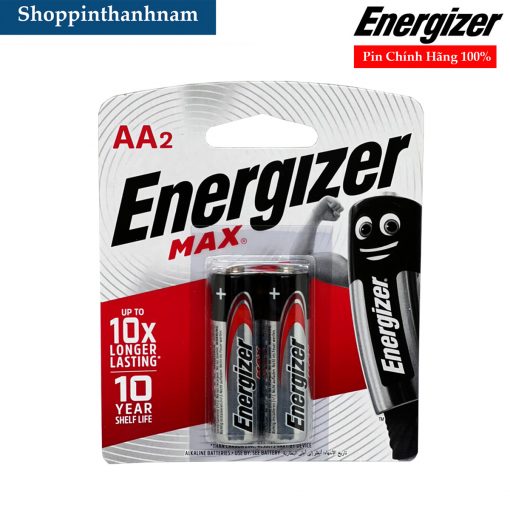In this image, the focal point is a digitally generated depiction of Energizer AA batteries in their retail packaging. Positioned in the top left corner is a dark blue rectangular button labeled "SHOPPINTHANHNAM" in white text. Adjacent to this button, on the right, is the brand name "Energizer" emblazoned in black font.

Beneath this, a bold red rectangle prominently displays the text "PINCHINH HANG 100%". The main section of the image showcases a front-facing view of the Energizer battery packaging, which features a light gray background. At the top of this packaging, the brand name "ENERGIZER" is prominently printed in black, with "MAX" inscribed in red just below it.

A playful logo of a battery character, flexing its arm, is present to the left side of the packaging. The character's arm is gray, and the battery body is black. Alongside this illustration, the packaging announces in white text, "UP TO 10X LONGER LASTING, 10 YEAR SHELF LIFE," set against a vibrant red background.

Additionally, there is a small hole towards the top of the packaging, typically intended for retail display purposes. The described elements collectively form a cohesive and detailed visual representation of the Energizer AA battery product.